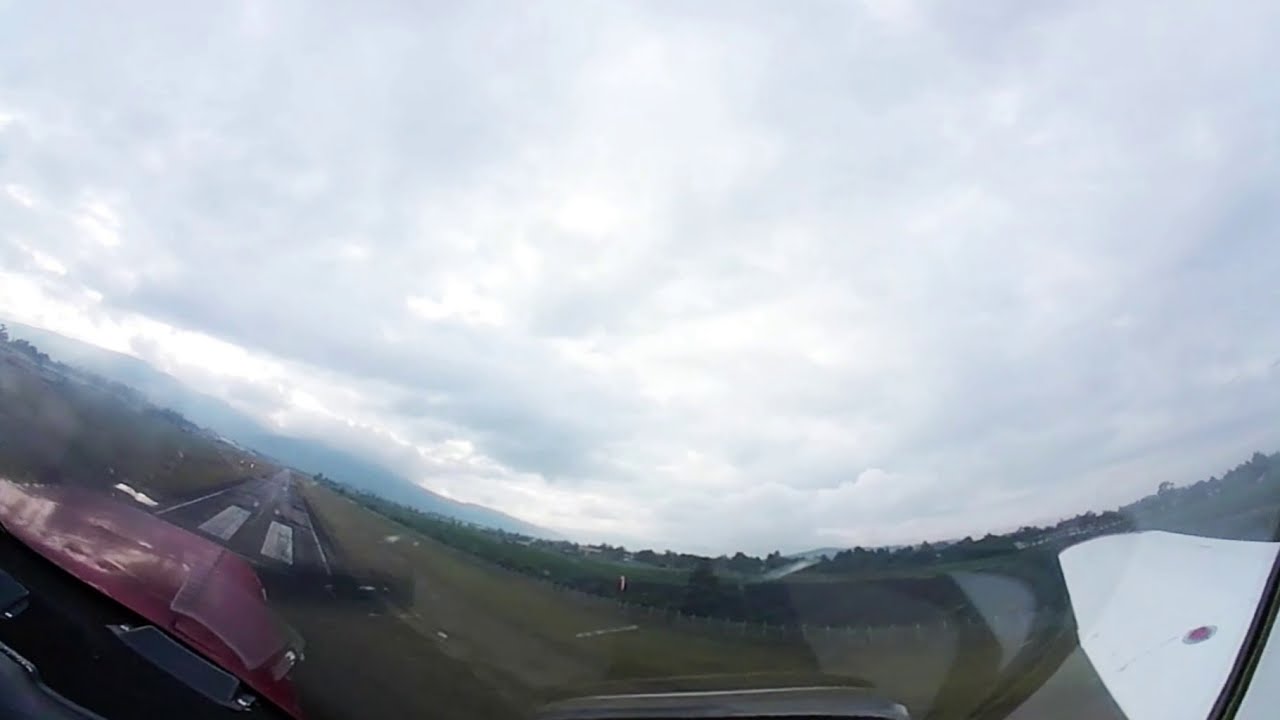This digital photograph captures a wide-angle view from inside the cockpit of a propeller plane, showcasing an expansive scene taken through a glass window. Central to the image is a clear runway, framed on both sides by vast, flat fields adorned with lush grass. The front of the plane, identifiable by its distinct red nose and the blurred, black movement of a propeller, suggests that the plane is either about to land or take off. Encircling the runway are open fields, stretching out to meet a dense forest along the horizon. The sky, dominating most of the photograph, is heavily overcast with thick, white clouds, casting a gloomy yet dramatic atmosphere. In the distant background, a range of mountains rises, adding depth and scale to the scene. The photograph's color palette includes hues of maroon, white, black, blue, gray, and green, enhancing the rich textures and elements within the frame. No text is visible within the image, maintaining its focus on the natural and man-made elements captured in this moment.